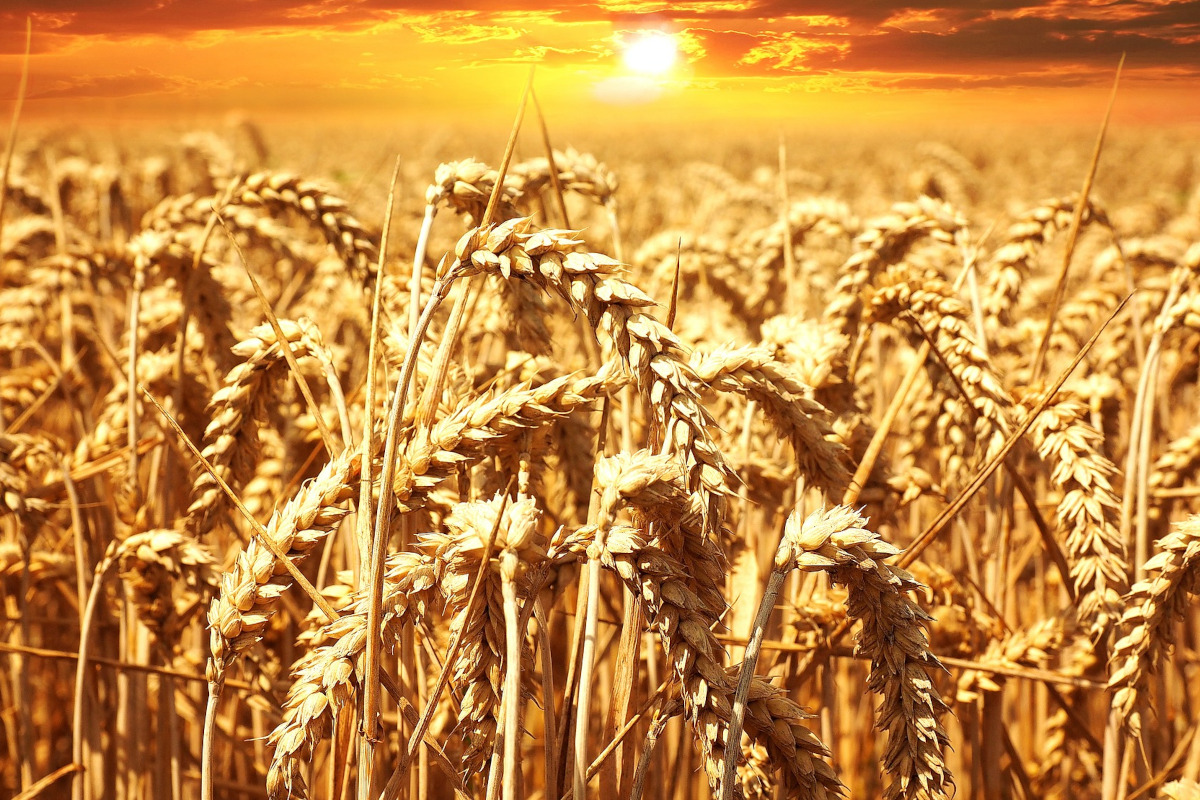This is a close-up, horizontal photograph of a serene wheat field taken outside during either sunrise or sunset. The forefront of the image showcases detailed wheat stalks with thin stems, topped with inch-long heads containing wheat grains that curl and droop gracefully. The field stretches into a vast expanse of wheat, fading into blurry, golden arches, indicating the vastness of the land covered in amber, yellow, and brown hues. The horizon reveals a striking sky painted in shades of orange, yellow, and golden, with the sun appearing bright white and casting reflections that create dark brown and burnt umber accents among the wheat. The upper part of the photograph features a golden sky adorned with soft clouds, emphasizing the enchanting beauty of the scene devoid of any landmarks, focusing solely on the wheat and the radiant atmosphere.